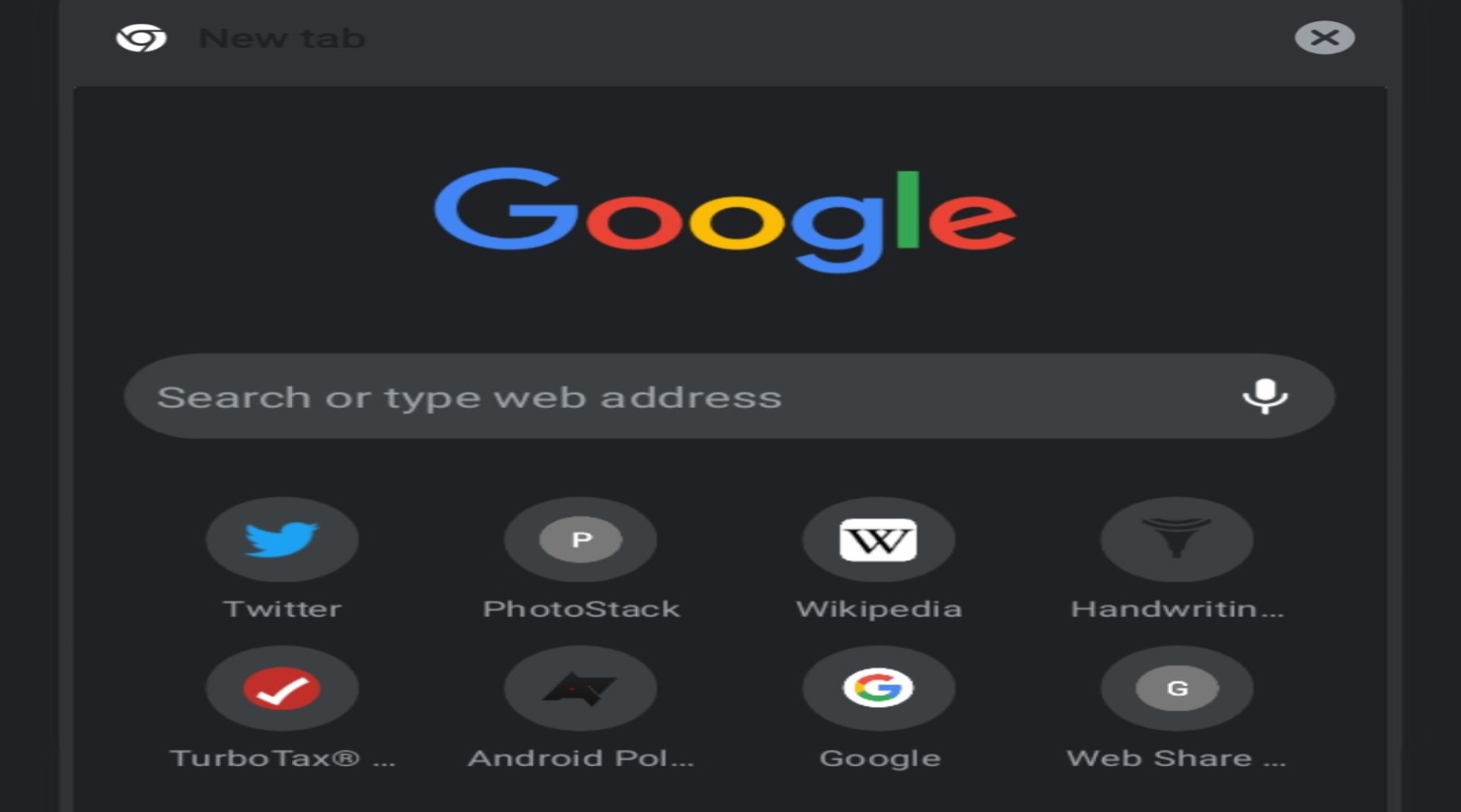The image captures a distorted screenshot of what resembles a Google search interface against a black background. The familiar Google logo is situated at the top, followed by the text "search or type web address." Below this, an array of icons representing various web pages or apps is displayed in two rows. Starting from the left on the first row, the icons are: Twitter, PhotoStack, and Wikipedia, with another icon resembling handwriting. The second row features icons for TurboTax, Android, P-O-L (indicating it might be truncated), Google, and WebShare. The overall appearance of the image is elongated and misshapen, suggesting that the screenshot may have been stretched or altered using photo editing tools.